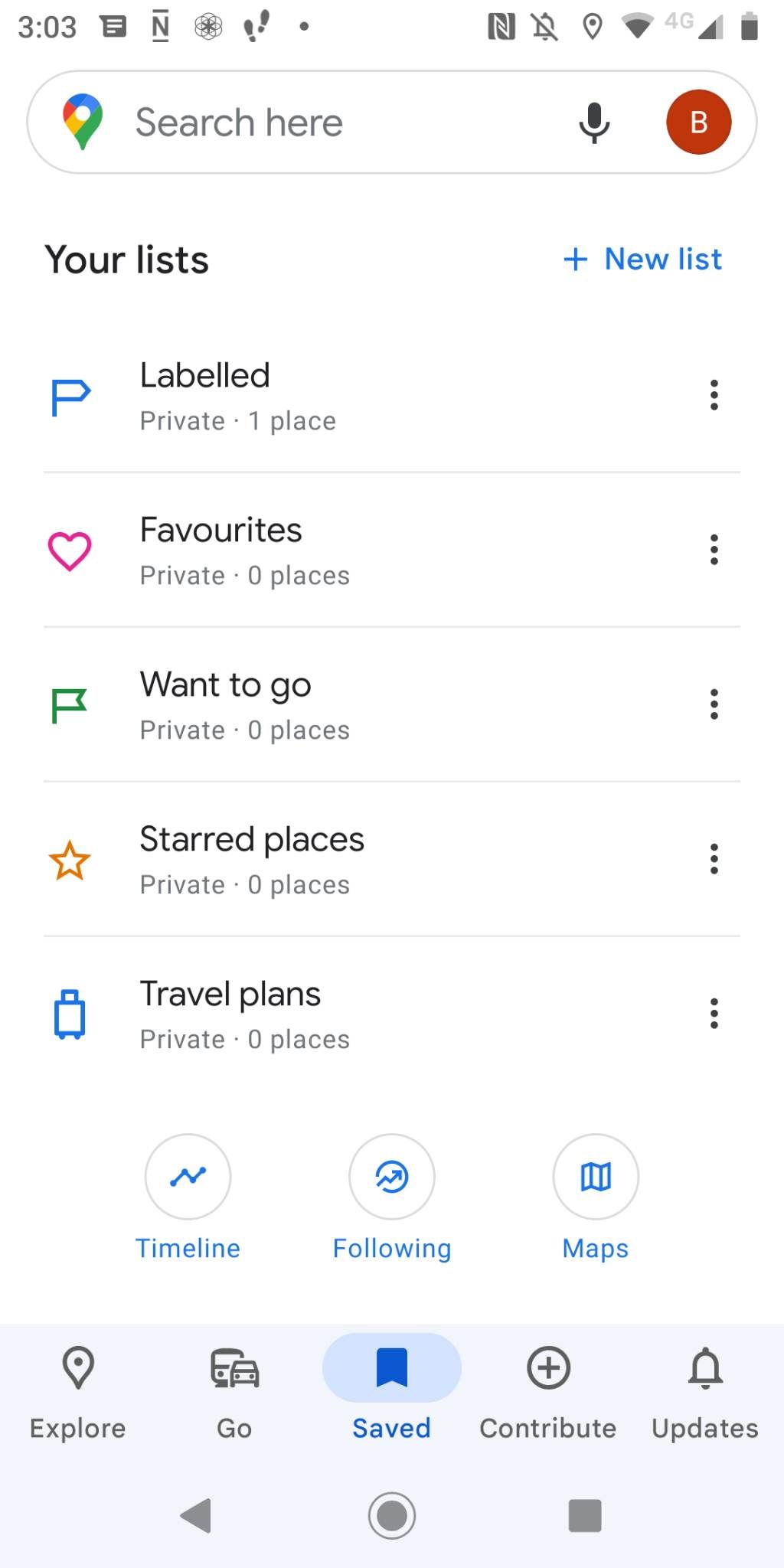The image depicts a smartphone screen in portrait mode with various UI elements, suggesting it might be part of an app for managing locations or lists. 

In the top left corner, the time is displayed as 3:03, accompanied by a text message icon labeled with an "N" between two lines. Adjacent to this, there is an icon resembling a footstep. On the right side of this top bar, a bell icon with a cross through it (indicating notifications are off), a marker icon labeled "that," and the typical reception, Wi-Fi, and battery icons are visible, with "4G" overlaid on the Wi-Fi signal.

Directly below this, a prominent white search box appears with text reading "Search here." To the right of the search box is a black microphone icon, a red circle containing a "B," and text reading "Your lists." Next to "Your lists," in blue, is the option to add a new list, labeled "+ new list."

Following this section is a series of tabbed lists, each labeled and color-coded:
- "Labeled" with various sub-items:
  - "Private: 1 place"
  - "Favorites: Private, 0 places"
  - "Want to go: Private, 0 places"
  - "Starred places: Private, 0 places"
  - "Travel plans: Private, 0 places"

Each of these items is accompanied by a corresponding color label.

At the bottom of the screen, three buttons are labeled "Timeline," "Following," and "Maps." Further navigation buttons below these options include "Explore," "Go," "Saved," "Contribute," and "Updates," likely offering additional features and functionalities within the app.